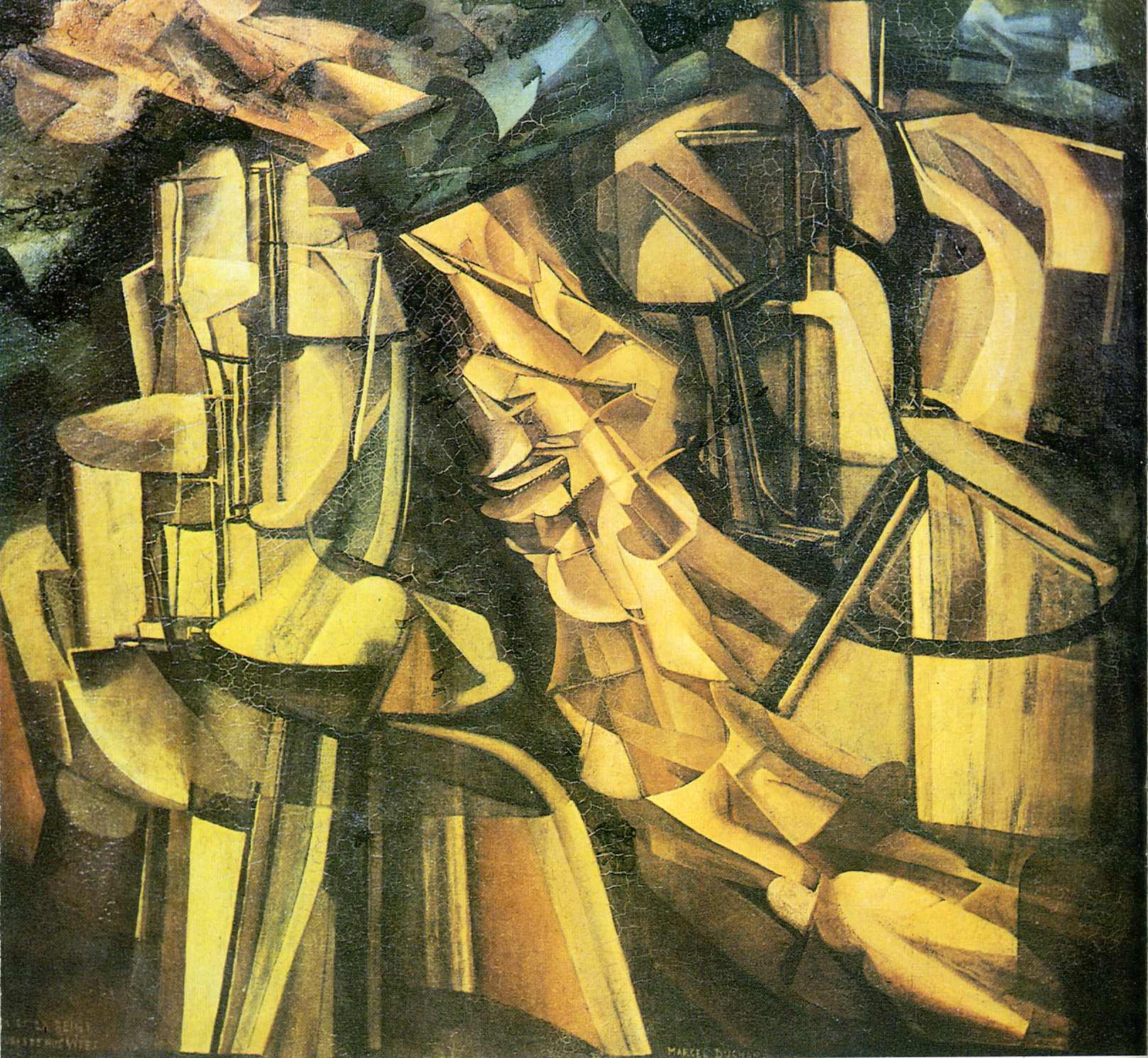The image is an abstract painting depicting a king and queen surrounded by swift lutes. The composition is complex, featuring a chaotic conglomeration of various abstract shapes and forms. Dominant colors include golden brown, yellow, black, orange, slate, and hints of green and light blue. The central focus of the image is a body formed from multiple abstract shapes resembling curved triangles and pie-like segments, predominantly in golden brown. Flanking this central body are yellow shapes composed of larger orange and black segments. The entire scene is an intricate blend of what appears to be mangled and strewn pieces of metal, suggesting a sense of entanglement and overlap. Despite the lack of textual elements, the painting's chaotic arrangement and diverse color palette capture a stunning yet bewildering abstract representation.